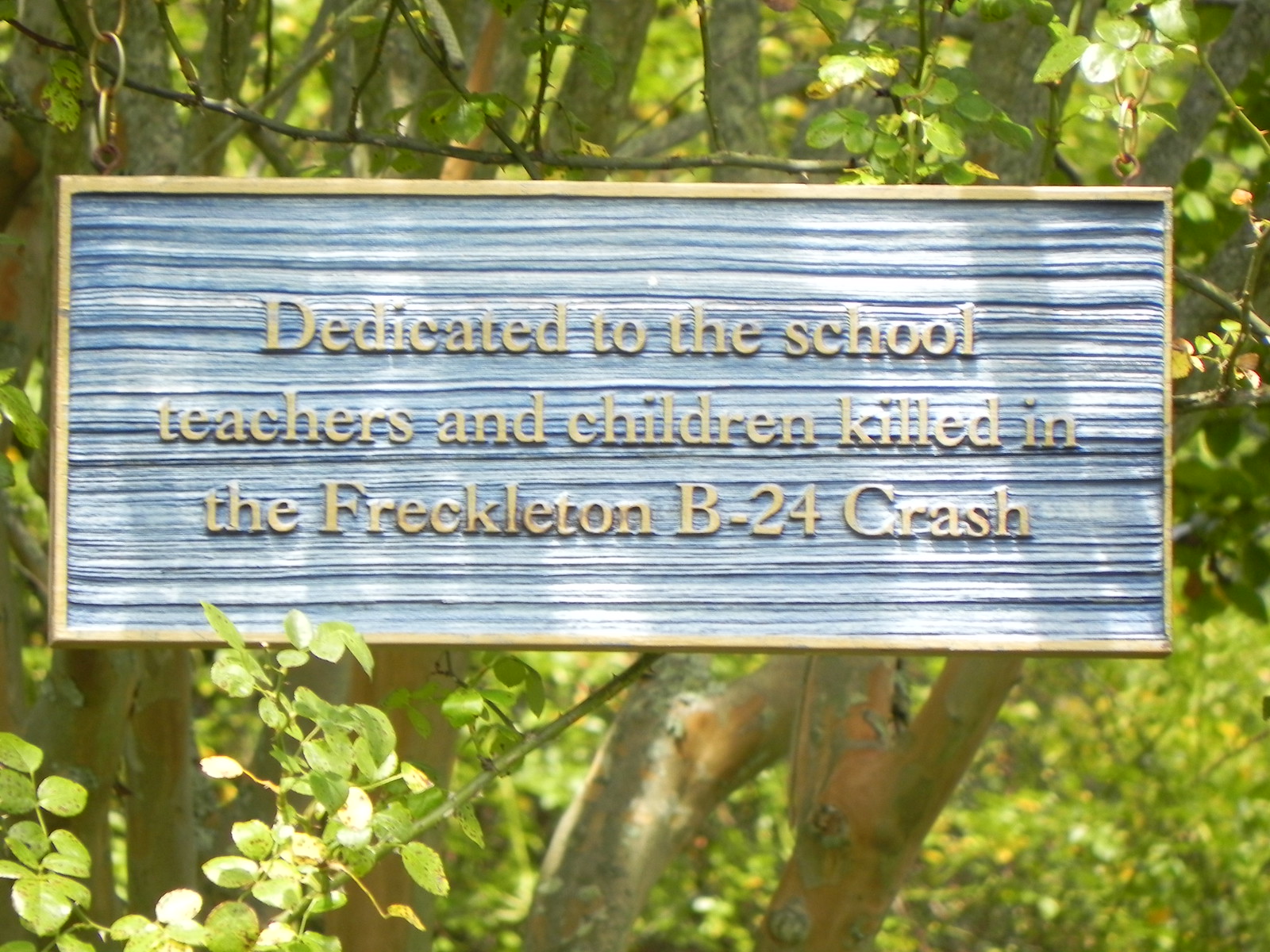In this full-color outdoor photograph, taken on a sunny day, a rectangular metal memorial plaque is prominently displayed, hanging from a tree by three gold-colored chains on each side. The tree behind the sign has lush green branches with small leaves, suggesting a densely wooded area. The plaque itself features a striking blue textured backdrop, creating an impression of washed blue metal, and is bordered by a matching gold frame. Centered on the plaque, embossed in gold letters, is the dedication: "Dedicated to the school teachers and children killed in the Freckleton B-24 crash." The sunlight highlights the verdant surroundings and the reflective qualities of the plaque, making it a poignant outdoor tribute.